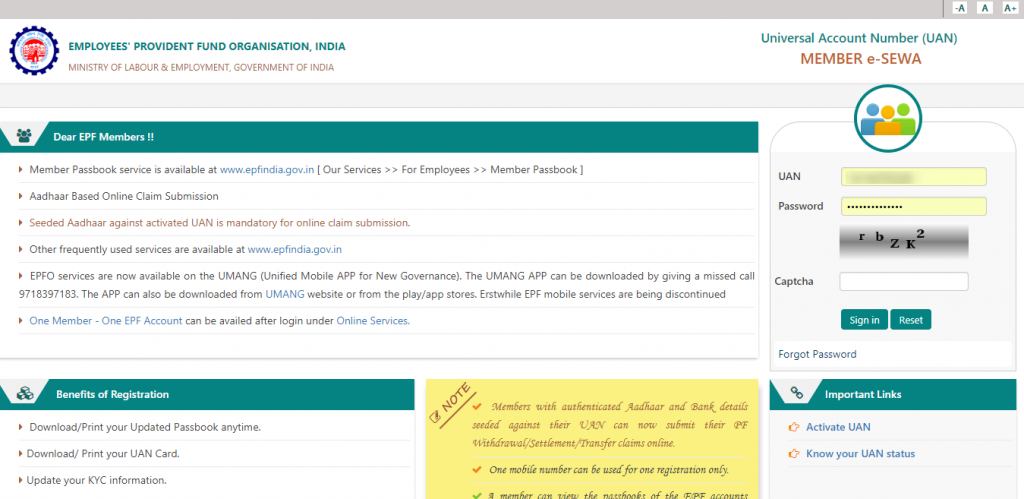The image depicts the homepage of the Employees Provident Fund Organization (EPFO) website in India. On the right-hand side of the webpage, there is a section labeled "Universal Account Number (UAN) Member e-Sewa." At the top left corner of the page, there is a small icon featuring a combination of blue, red, and white colors. The page displays two prominent green banners: the first one addresses EPF members with the message "Dear EPF members," and the second one lists the "Benefits of Registration."

To the right of these banners is a login area where users can enter their UAN and password. This section also includes a CAPTCHA, which currently reads "RBZK2," as well as green "Sign In" and "Reset" buttons. There is also a "Forgot Password" option available below the login inputs.

Beneath this, a long green rectangular box labeled "Important Links" is present. This section includes hyperlinks identified with small orange hand icons: "Activate UAN" and "Know Your UAN Status." Finally, at the very bottom of the page, there is a yellow box with cursive text discussing mobile numbers and their usage related to member accounts.